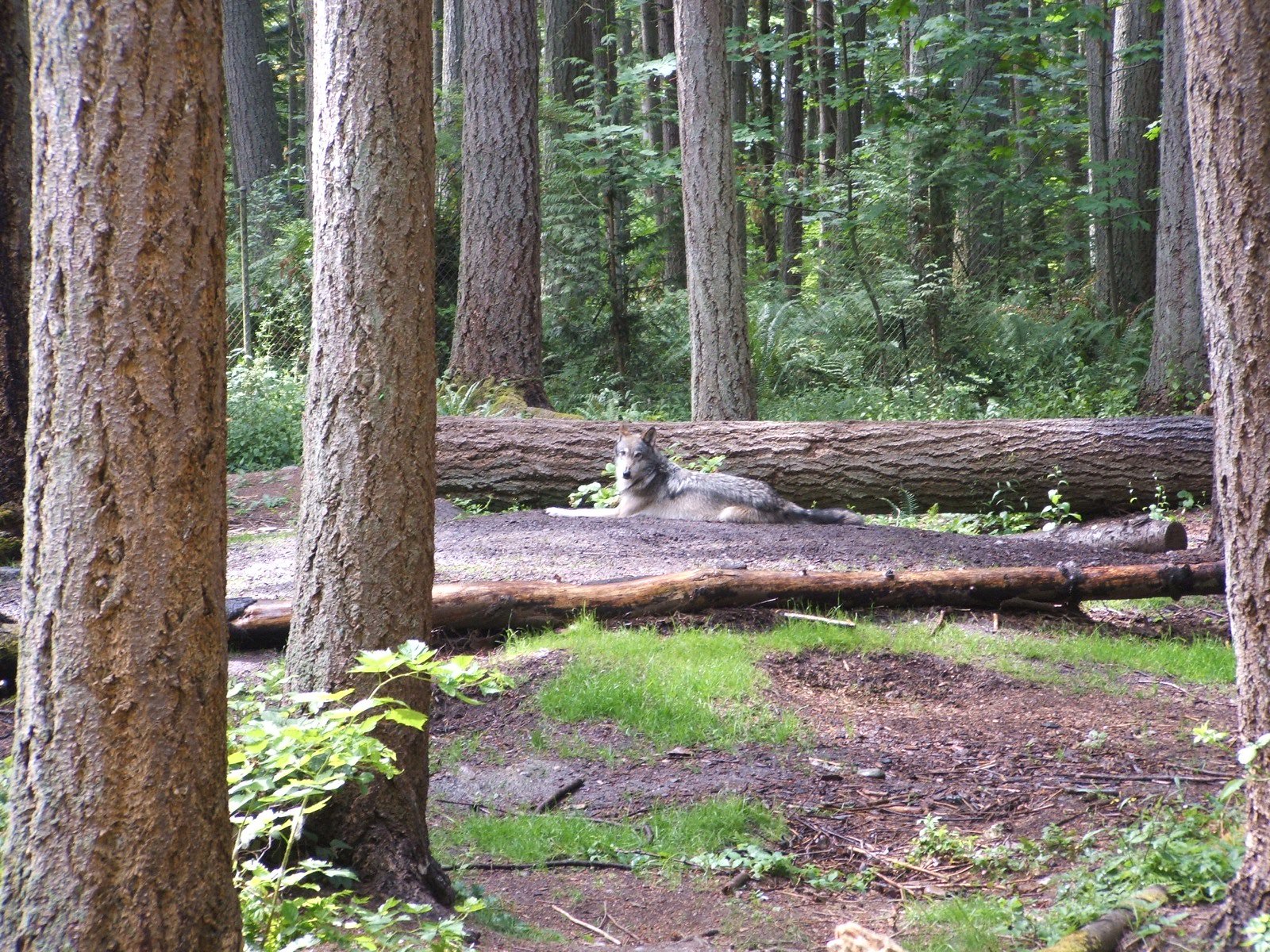In this detailed forest scene, the photograph captures a tranquil woodland setting with a multitude of towering trees rising from the dirt and grassy ground. The trees, predominantly green with brown bark, form a dense backdrop, interspersed with smaller shrubs and greenery. Prominently in the center, a gray wolf lies stretched out on the forest floor, with its legs and tail extended, gazing directly at the camera. The wolf's fur exhibits a mix of white and black, contrasting with the earthy tones surrounding it. Adjacent to the wolf are two large horizontal tree trunks, one partially cut out, adding an element of natural ruggedness to the composition. The dense concentration of approximately six towering tree trunks frames the scene, encapsulating the serene and wild essence of the forest.